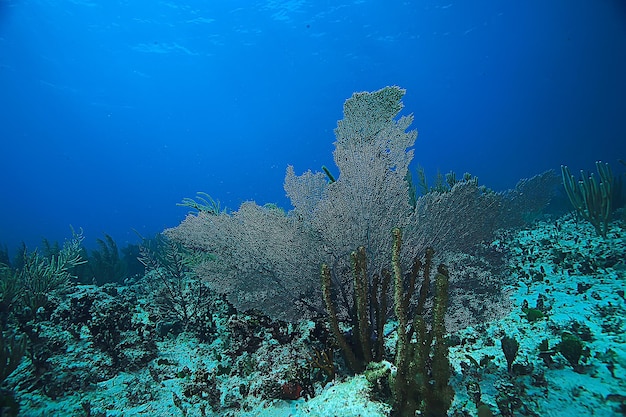This photograph captures an underwater scene rich with oceanic life and color. The background is a deep blue, punctuated by ripples of sunlight filtering down from the surface, giving a serene, almost royal blue hue to the entire image. The foreground showcases the ocean floor, covered in sandy hues that blend into blue and green due to the lighting. A sprawling coral reef dominates the scene, adorned with various corals and plants. In the center, the focal point is a large, leaf-shaped coral in a striking white or light gray color. Surrounding it are numerous smaller corals, varying in shape and color, including finger-like and cactus-shaped formations in shades of green and yellow. This vibrant underwater tableau is a harmonious blend of coral structures and marine flora, highlighted by the interplay of natural light and oceanic hues.